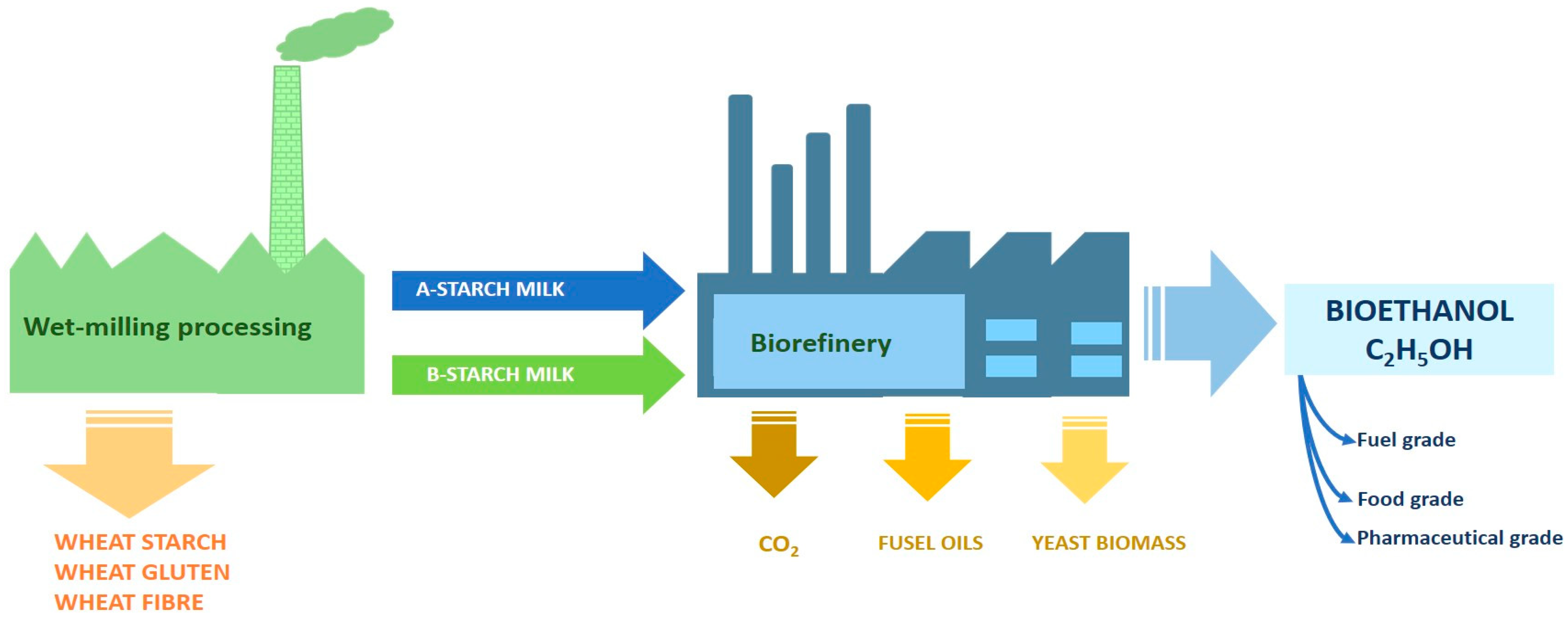The image is a detailed graphic illustrating the bioethanol manufacturing process through wet milling processing. It features an outdoor setting with a green plant or smokestack emitting smoke. The graphic text begins with "wet milling processing," followed by a downward-pointing yellow arrow marked "wheat starch, wheat gluten, wheat fiber." 

To the right of this, two arrows (one blue and one green) labeled "starch milk A" and "starch milk B" respectively lead to a larger plant or refinery with four smokestacks, signifying a biorefinery. Within this biorefinery section, there are arrows pointing downward labeled "CO2," "fusel oil," and "yeast biomass."

Furthermore, a blue arrow leads to a blue box labeled "bioethanol, C2H5OH." This box has further blue arrows pointing downward, specifying different grades of the produced bioethanol: "fuel grade," "food grade," and "pharmaceutical grade." The entire diagram captures the step-by-step transformation from raw wheat components to various grades of bioethanol.